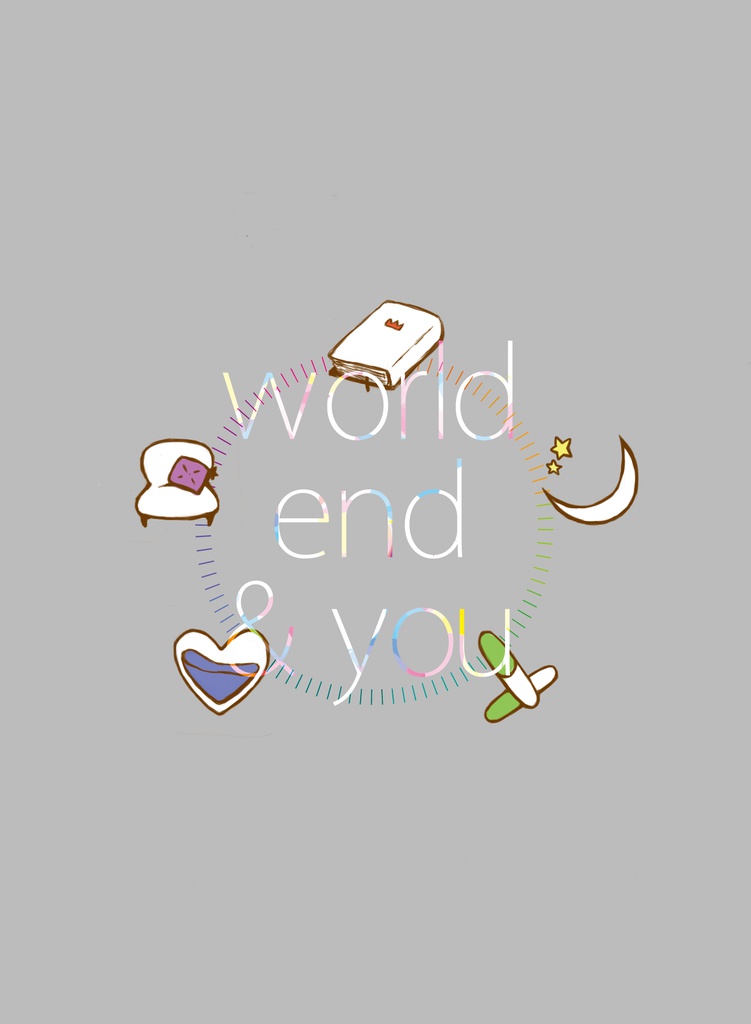The image features a digital design set against a solid gray background. Central to the image are the words "world," "end," and "you," written in a dynamic, rainbow gradient that shifts colors throughout the text. Below the text, multicolored lines intersect to form a circular pattern, transitioning through green, blue, and other hues as they complete the circle. Surrounding this circle are illustrations of various objects: a closed white book with a red crown atop it at the top, a crescent moon with two yellow stars to the right, two capsule pills—half green, half white—in the bottom right, a white heart filled with blue liquid splashing about in the bottom left, and a white sofa chair with a pink cushion on it towards the top left. The entire composition brings a rich array of colors and intricate details against the minimalist gray backdrop, offering a visually engaging and complex design.